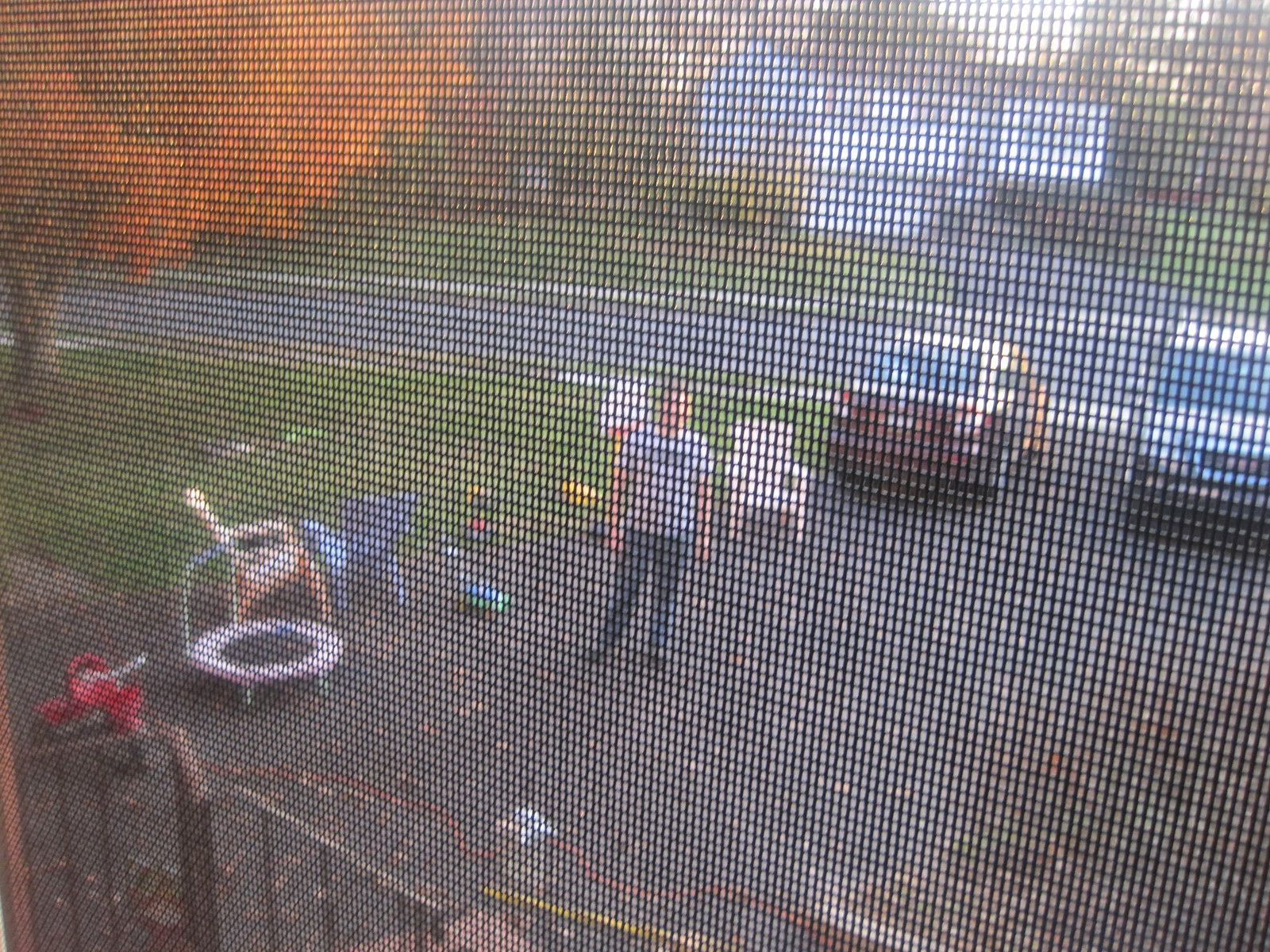In this photograph taken from behind a screen door or a screened-in patio, a faint black mesh pattern overlays the entire image. The scene reveals a gray paved driveway adjacent to a house. Standing in the driveway is a man wearing a white shirt and blue jeans. The driveway accommodates two vehicles: a gray SUV and a red car.

Scattered around the driveway are various objects, including a white patio chair and a pair of colorful patio chairs—one blue and the other orange. A pink exercise-style trampoline with a support bar stands near the center of the image, accompanied by a red tricycle designed for a small child. The ensemble of items lends a casual, lived-in feel to the scene, giving a glimpse into a typical, everyday setting.